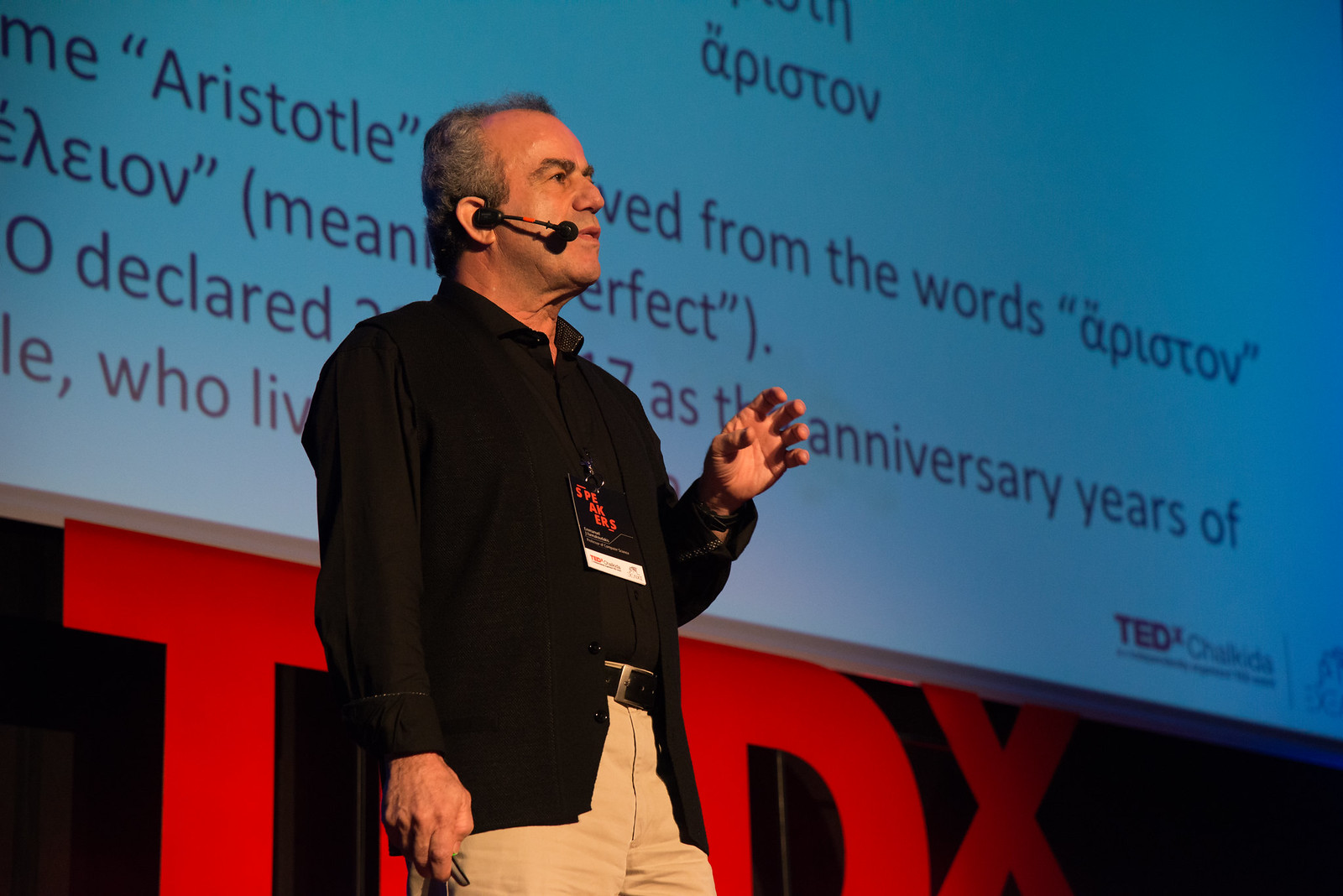The detailed photograph depicts a middle-aged man, likely in his 50s, delivering a TEDx talk. He stands on a stage adorned with the recognizable TEDx branding in bold letters behind him. His attire includes a black suit jacket over a black button-up shirt, paired with tan chinos. He is equipped with a small, cordless hands-free microphone that wraps around his right ear, suggesting a professional setup commonly used in presentations.

The man is positioned to the left of the image, captured in a moment of speech while making a gesture with his left hand. His partially balding hair is graying, adding to his distinguished appearance. The photograph, likely taken by a professional given its clarity and texture, shows him looking to his right, engaging with the audience off-screen.

Behind him, a large screen displays fragments of text in both English and another language that appears to be Greek. The screen includes words like "Aristotle," "declared," and "perfect," and partial phrases such as "derived from the words" and "the anniversary years of," suggesting a discussion that delves into historical or linguistic topics. The well-lit scene and the man's composed demeanor encapsulate the essence of an insightful TEDx presentation.